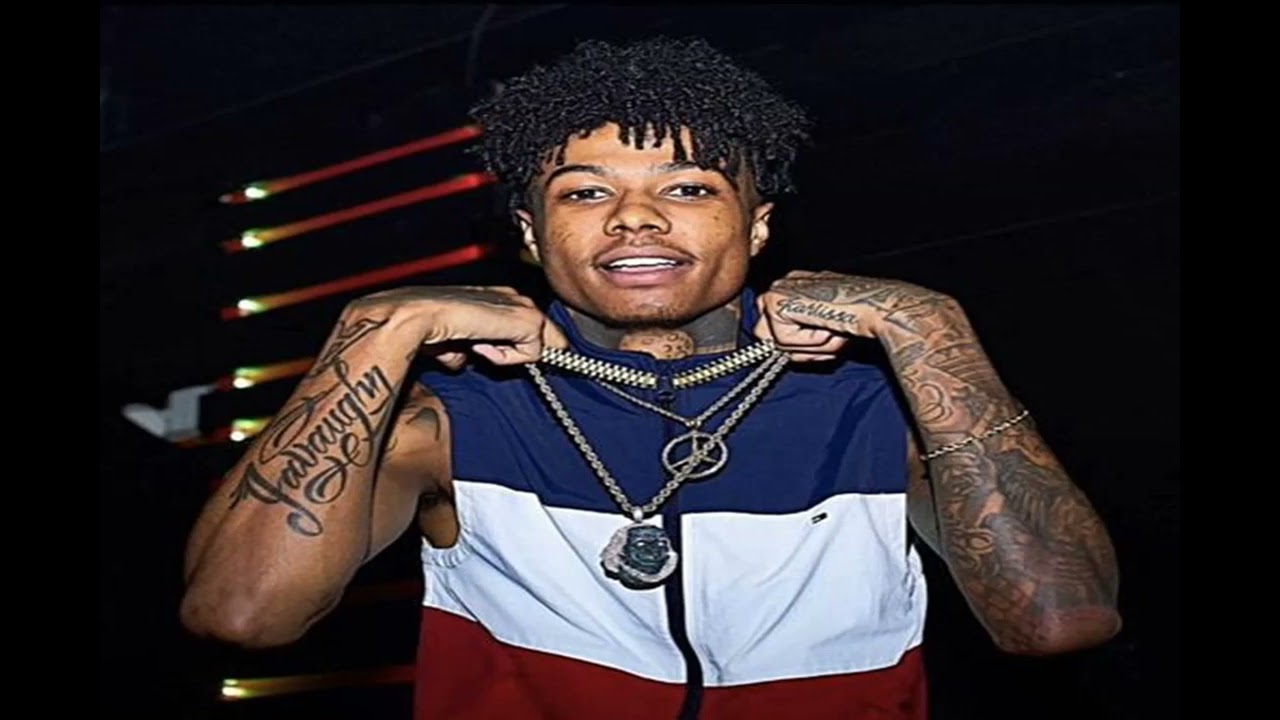The image features a young black man with medium-length curly hair, smiling broadly at the camera, exposing both his upper and lower teeth. He is centered against a predominantly black background with decorative orange ambient lighting on the left side, resembling bars or club lighting. The man is dressed in a distinctive sleeveless zip-up vest with a blue top, white center, and red bottom. He's holding up two necklaces, one featuring a Mercedes-Benz logo and the other displaying a blinged-out face of Benjamin Franklin. His right arm shows a tattoo in cursive black text that reads "Javaughy," while his left arm bears another tattoo that says "Carlissa." Additionally, he has a flower tattoo on his neck and wears a bracelet on one wrist. The detailed tattoos covering his arms and his fashion sense suggest he might be a rapper.